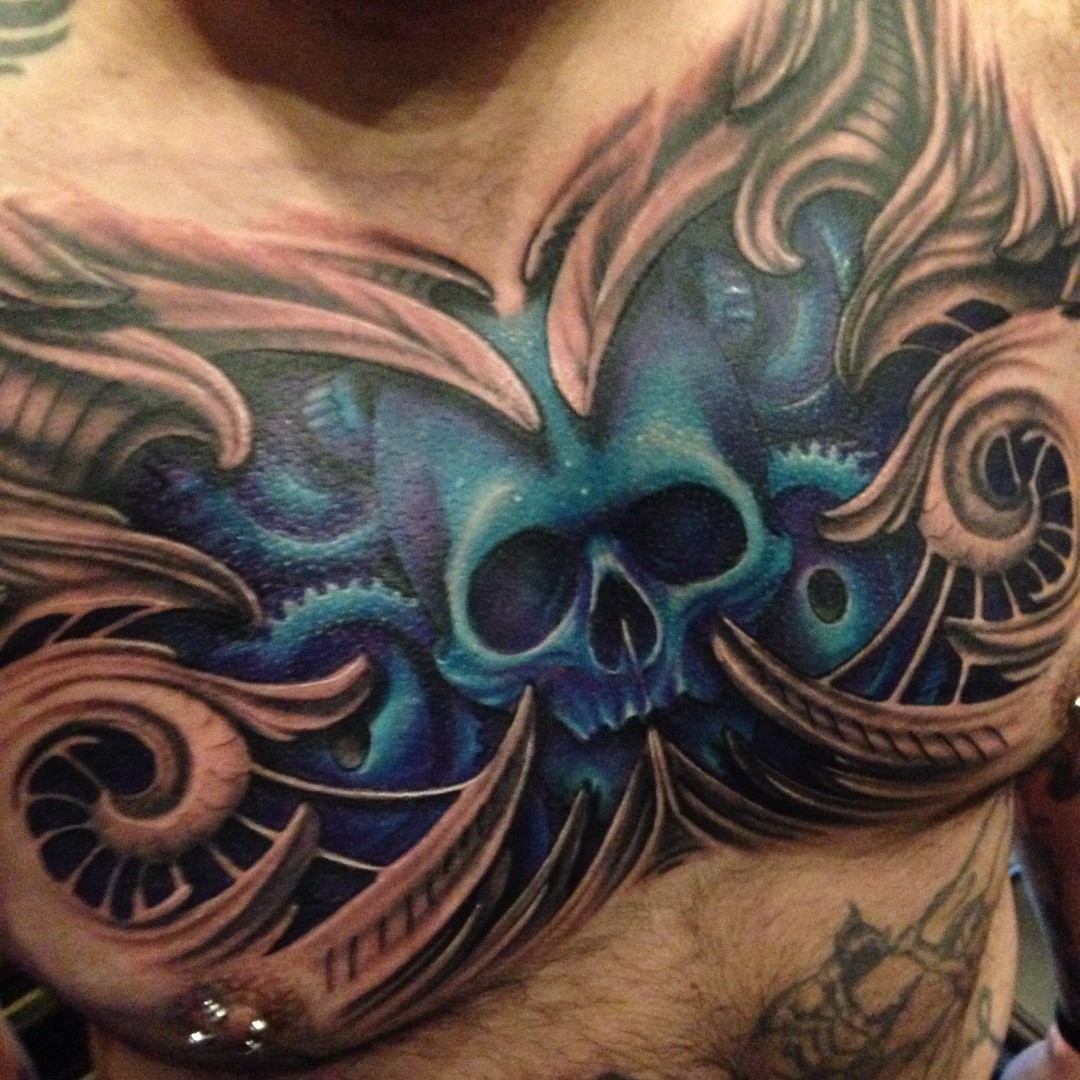This image features a close-up view of a man's chest adorned with extensive tattoos. The central focus is a detailed tattoo of a human skull, which is a dark purplish-blue color and lacks a lower jaw. The skull's hollow eyes and nose are prominent against his skin. Surrounding the skull are curly, spiral-shaped designs resembling octopus tentacles in a mix of bluish-purple and reddish-beige hues, with some black accents. Additionally, the man has silver nipple piercings. The photograph captures the area from just below his neck to slightly below his chest, with partial visibility of another tattoo near his belly button. His chest also has some black body hair.